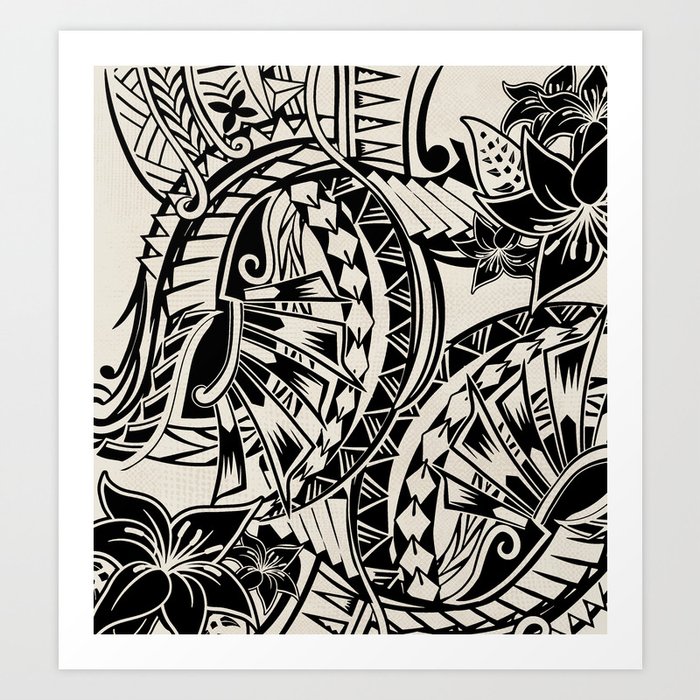The image is a highly detailed, abstract graphic rendered in a black and white, vector style. It resembles a photograph or framed picture with a distinct white border, placed against a gray background. The overall composition is complex, with a multitude of geometric shapes including numerous triangles, rectangles, and diamond-like patterns. Central to the design are several black hibiscus flowers; one prominently located in the bottom left corner featuring white stamens, and a few others visible in the top right corner. These flowers are characterized by their black petals and contrasting white edges. Amidst these floral elements are tribal-like, Hawaiian-inspired designs, with large swirls and intricate patterns that add to the overall abstract nature of the image. The imagery is primarily in tan and black, making the bold geometric and tribal motifs stand out against the background.